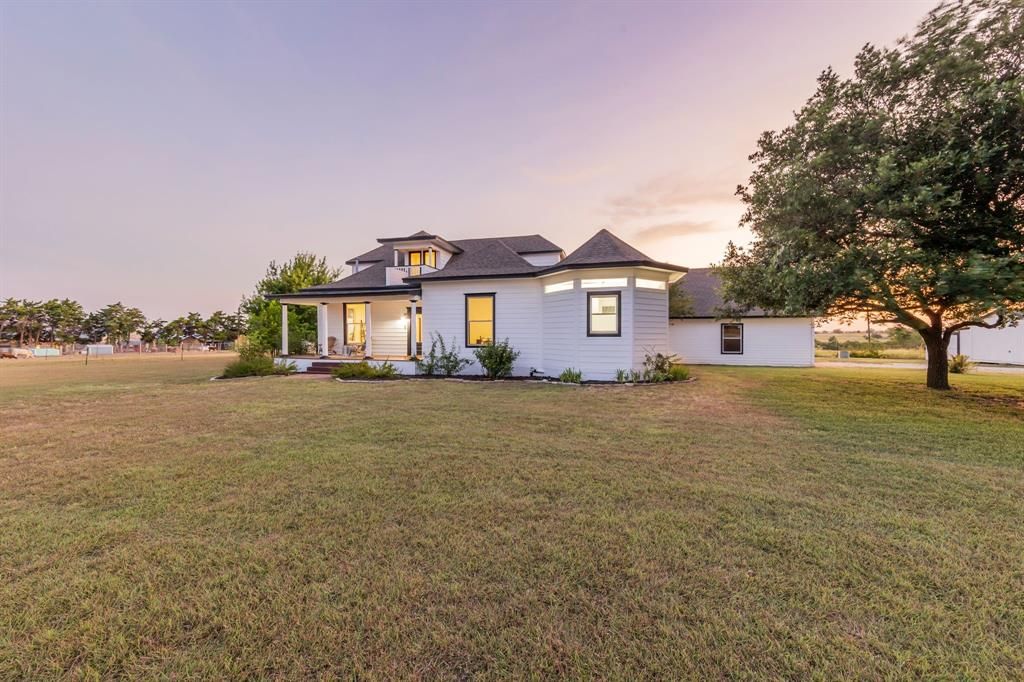The image showcases a solitary white house with horizontal siding, nestled in a well-manicured lawn displaying some green and graying patches. The house, illuminated by a warm amber glow from its numerous windows, stands prominently beneath a captivating sky transitioning from deep purple to blue with hints of yellow and red, indicating dusk. On the right side of the house extends a white garage, and there's a distinct hexagonal-shaped room with a matching roof that ascends to a triangular point. Above the main structure, a second-floor porch is supported by four white pillars. A sprawling green lawn, approximately an acre in size, stretches out in front of the house, dotted with a garden bed bordered by rocks. To the right of this serene scene, a deciduous tree with a short brown trunk extends upward, while a driveway stems from the garage, leading out of the frame. In the distance, a fence line and additional trees frame the view, with a few scattered buildings peeking through, complementing the peaceful rural setting.